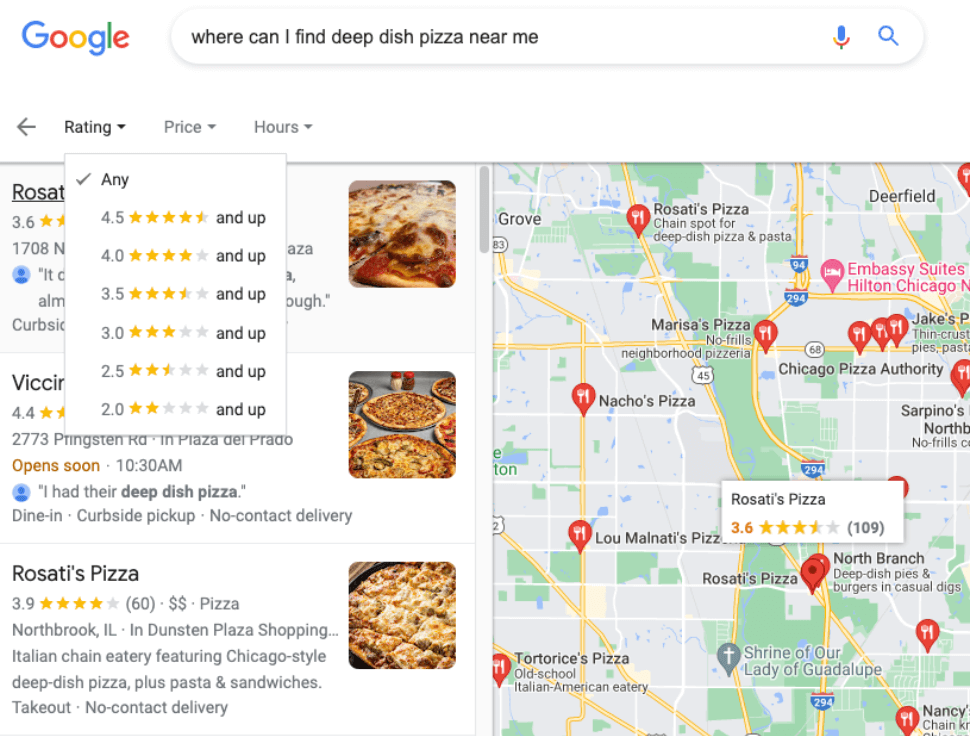This image is a detailed screenshot from a Google search results page. The background is predominantly white. In the upper left-hand corner, the Google logo is prominently displayed, featuring a blue "G," a red "O," a yellow "O," a blue "G," a green "L," and a red "E." To the right of the logo is a search box showing the query, "where can I find deep dish pizza near me?" in gray font.

On the left side of the page, there are listings for three pizzerias, each accompanied by a small photo. The first listing features a close-up image of a single slice of pizza. The second listing showcases an overhead view of two full pizzas and parts of two others. The third listing includes a top-down view of a whole deep dish pizza. The most visible listing in the lower left-hand corner has the name "Rosati's Pizza" with a star rating of 3.9.

To the right of these listings is a detailed map focused on the Chicago area, highlighting various pizza restaurants with red teardrop-shaped markers. This map provides a close-up view of the greater downtown area of Chicago.